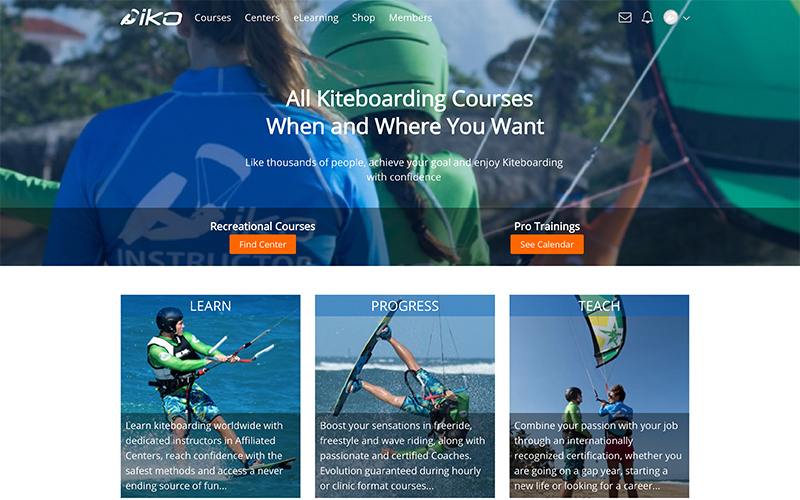Screenshot of the desktop version of a website showcasing kiteboarding activities. At the top of the page, there's a navigational menu with a semi-transparent background overlaying an image of people kiteboarding. The menu features the iKO logo on the far left and white text options for "Courses," "Centers," "E-Learning," "Shop," and "Members." 

Centrally located, a prominent headline reads: "All Kiteboarding Courses, When and Where You Want." Beneath this headline, there is a smaller text stating, "Like thousands of people, achieve your goal and enjoy kiteboarding with convenience."

Further down, two clickable buttons are visible: "Recreational Courses" with a "Find Center" option and "Pro Trainings" accompanied by a "See Calendar" option.

Below these buttons, three smaller clickable rectangles are displayed in a row, each containing an image with overlaid text. The first rectangle, labeled "Learn," the second, "Progress," and the third, "Teach," all feature images of individuals engaged in kiteboarding activities.